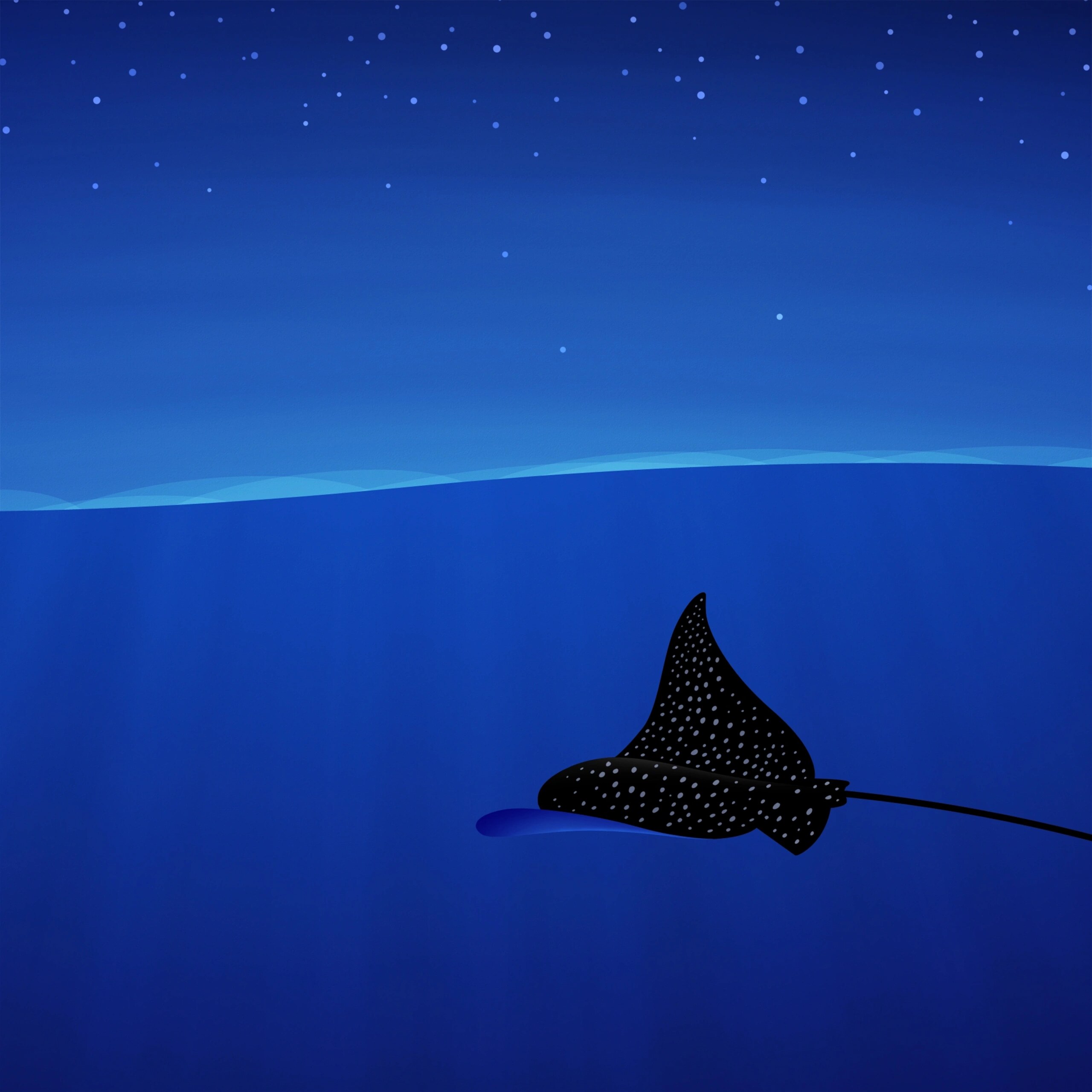This image showcases a surreal, possibly digitally generated painting of a large black stingray gliding through the ocean beneath a night sky. Rendered in a minimalist style with limited colors, the backdrop transitions from a lighter blue at the horizon line to a deeper blue, signifying the depths of the ocean. The horizon is depicted as a thin, bright aqua blue line dividing the sky and water. The sky above is adorned with light blue dots representing stars. The black stingray, positioned in the center right of the image, features white spots adorning its body and a long, stinger-like tail. The overall composition suggests an abstract representation of an underwater scene, with elements hinting at a dreamlike or fantastical quality.